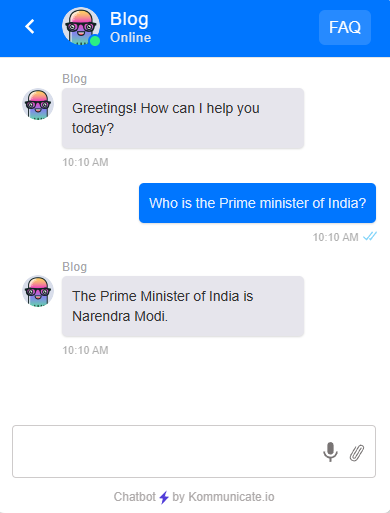This image depicts a snapshot of an online blog conversation, identifiable by a royal blue header at the top labeled "Blog Online." The header features a cartoonish avatar resembling an octopus-like creature with small tentacles, wearing glasses, and possessing a beak-like area. A green dot near the avatar indicates the user is online. Adjacent to this, the text "Blog Online" is prominently displayed, along with an "FAQ" label at the far end.

In the conversation section, the user on the left initiates with "Greetings, how can I help you today?" timestamped at 10:10 a.m. The response appears in blue text on the right, asking, "Who is the Prime Minister of India?" at the same time, 10:10 a.m., marked by two blue check marks indicating the message has been read. The left side of the blog then replies, "The Prime Minister of India is Narendra Modi."

Below the conversation, there is a text input field labeled "Chat box by communicate.io" where users can type their next message. The setup of the conversation window is clean and straightforward, facilitating easy navigation and interaction for users.